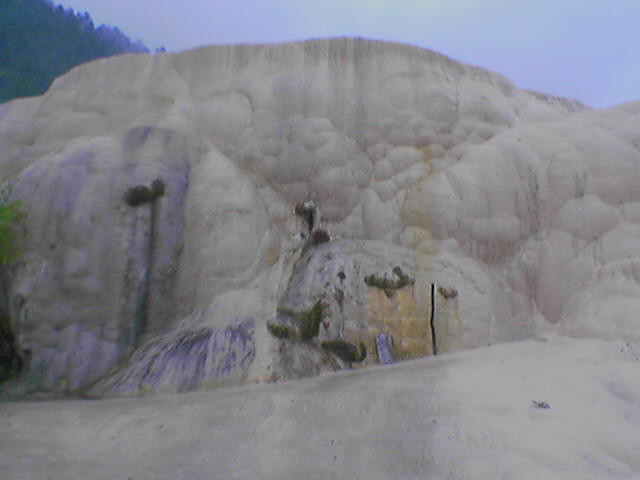This image depicts a rocky mountainside dominated by a light beige sandstone or limestone formation that occupies the majority of the frame, approximately 95%. The rock surface appears puffy and billowy, reminiscent of white clouds, yet detailed with darker splotches and streaks in various hues, including black, pale orange, dark gray, and deep purple. Towards the bottom, some blue lines are visible, adding to the contrasting array of colors. The photograph, though grainy and possibly taken under low-light conditions or with an inferior camera, captures some greenery and vegetation situated in the upper left corner, suggesting a mountain environment. The sky at the top of the image is a faint shade of blue, slightly overexposed, with an indistinct presence of cloud cover. The scene is entirely devoid of people, buildings, or vehicles, focusing solely on the natural landscape.